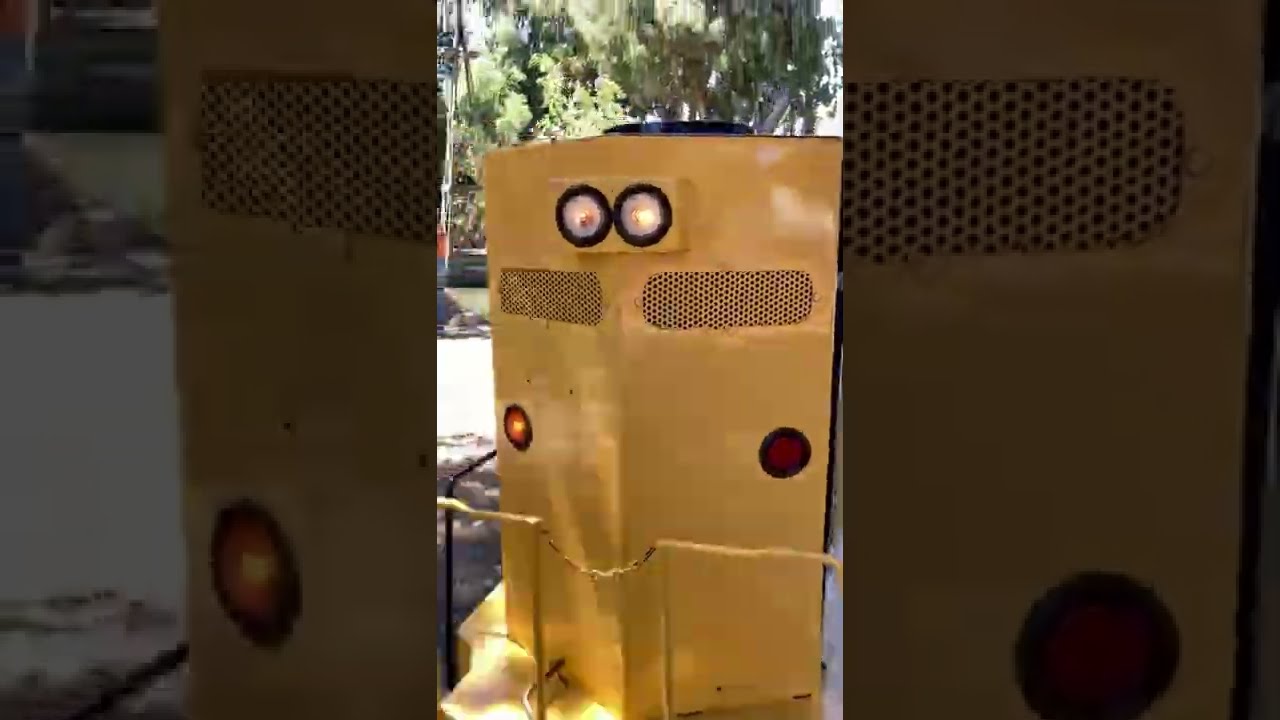The image depicts a yellow piece of machinery, possibly the rear or engine of a small amusement park train. It has a distinct rectangular shape that tapers inward slightly in the middle, giving it a somewhat half-triangle appearance. The device is outdoors on a sunny day, evidenced by the trees visible in the background. The structure features a yellow metal frame that resembles a fence line at its base. The top part of the machinery includes a rectangular box with two white lights, and below that, there are two round orange lights close together. Further down, it has two red lights positioned apart from each other, and just above them are pill-shaped grills. The machinery seems like it could be a small train car meant for children’s rides, rather than a full-sized train, possibly found in an amusement park or similar setting.